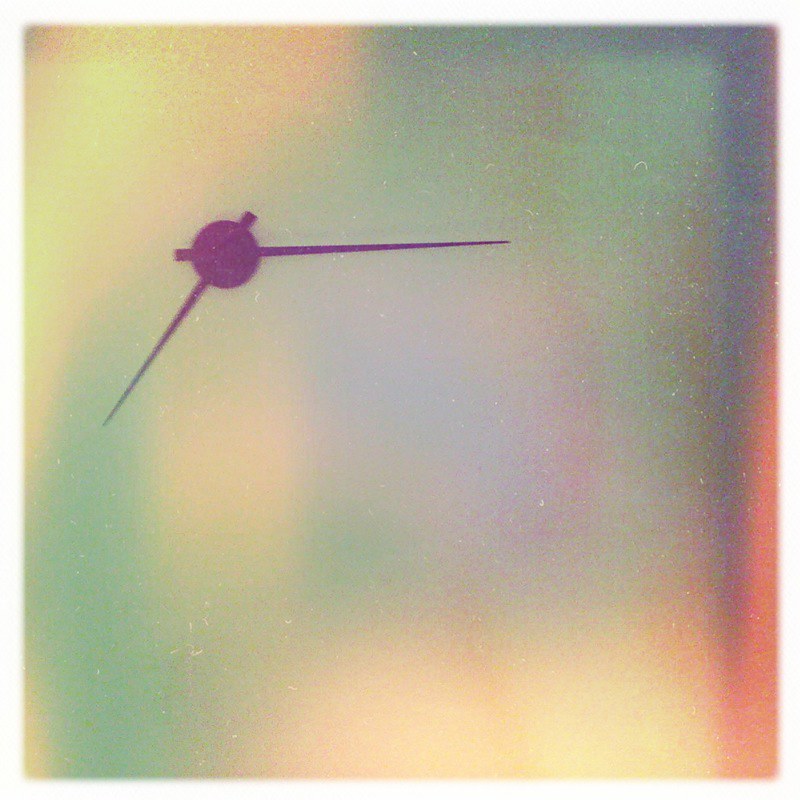This image is a square digital artwork with fuzzy edges and rounded corners, possibly featuring a very subtle white trim. The dominant colors are yellow and green, creating a gradient of shades across the image. In the top left and bottom right corners, there are brighter, yellowish-white areas that appear lit. Centrally, purplish-green hues blend from the top right to the bottom left. A purple circle, just down from the top left, marks a focal point. Emerging from this circle are two thin, black hands resembling those of a clock: one extends from the top right towards the left, indicating roughly 5:14, while the other stretches from the top left downwards to the right. Additional accents include a bright orange band near the middle, and subtle blue and red tinges along the edges, contributing to the artwork’s vibrant and abstract nature.